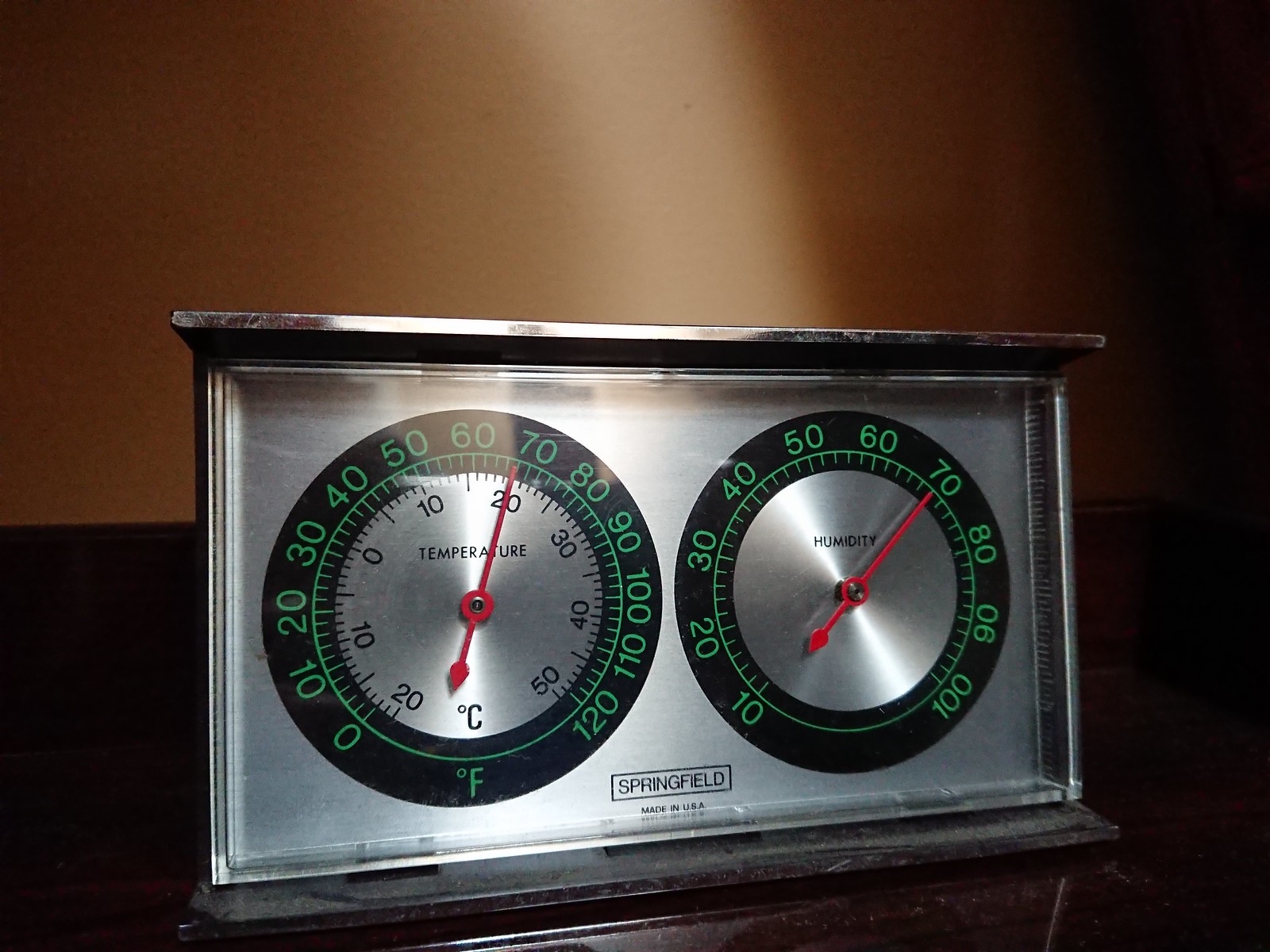In this detailed photograph, there is a temperature and humidity gauge placed on a dark mahogany wood surface. The background wall is textured and painted a deep orange color. The device appears to be made of either chrome plastic or actual chrome, with a clear plastic cover protecting the dials. 

The gauge has two circular dials side by side. The left dial is marked "Temperature" and features both Fahrenheit and Celsius scales. The outer green scale for Fahrenheit ranges from 0 to 120 degrees, while the inner scale for Celsius ranges from -20 to 50 degrees. The current temperature is indicated by a red pointer, which shows 69 degrees Fahrenheit and 20 degrees Celsius.

The right dial is labeled "Humidity" and displays a range from 0 to 100 percent. The red pointer on this barometer is currently indicating a humidity level of 70 percent. The face of the device is labeled "Springfield" and "Made in the USA" in small lettering.